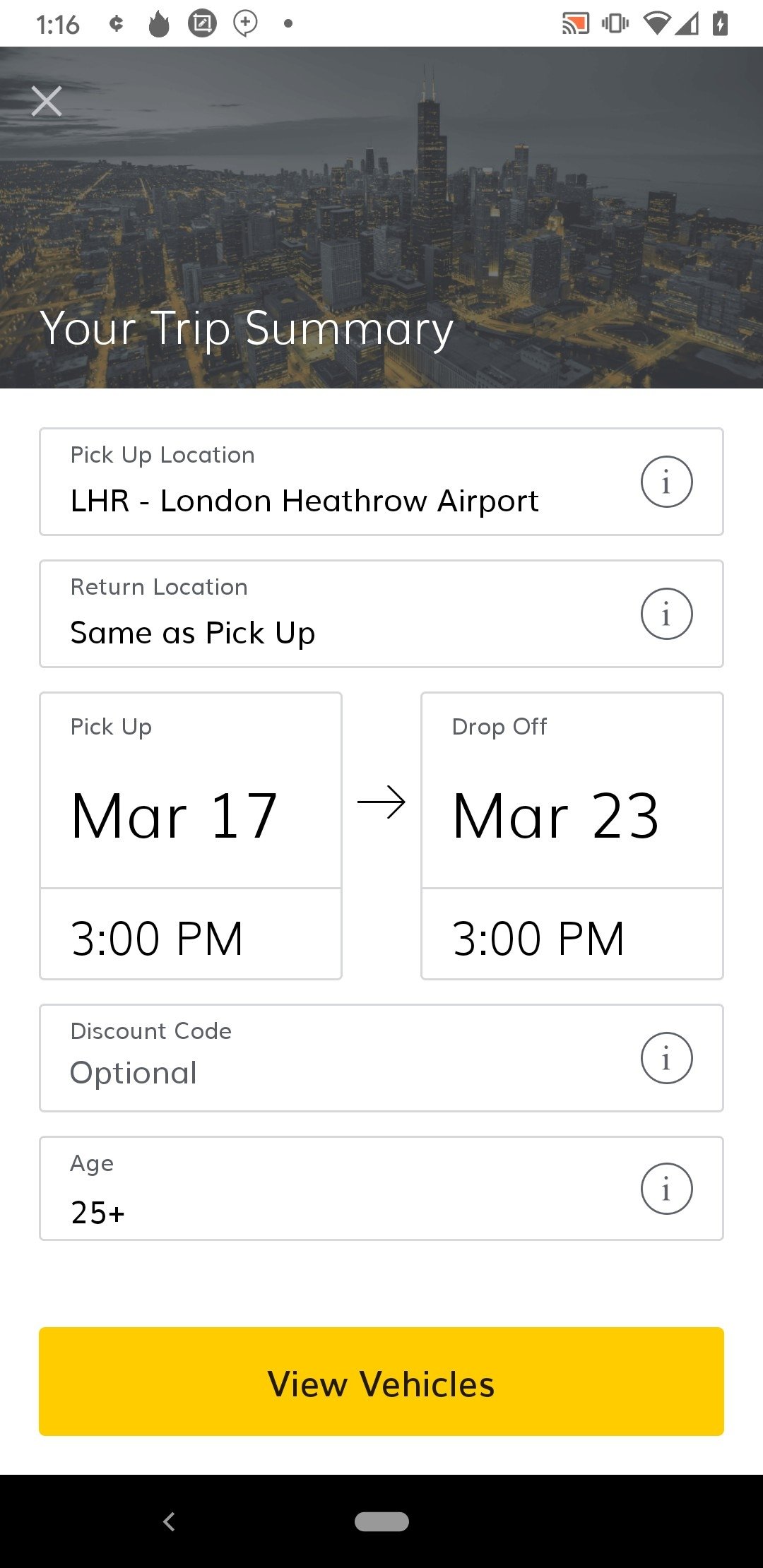In this detailed screenshot from a mobile phone, we observe what appears to be a travel app interface. The phone status bar at the top indicates the device's current status—it shows the time, the screencast icon, the vibrate mode being enabled, Wi-Fi signal strength, battery level, and network signal strength.

The main content begins with a visually engaging picture of a sprawling metropolis, labeled with an "X" in the corner, indicating an option to close the image. Underneath the image, a title reads "Your Trip Summary," suggesting that this section outlines the key details of the user's travel itinerary.

Further down, there's a segmented bar designating the "Pickup Location" as "LHR London Heathrow Airport," accompanied by an information button for additional details. Similarly, "Return Location" is noted as "Same as Pickup," also with an accompanying information button.

A larger box beneath these details presents the pickup and drop-off dates and times: "Pickup, March 17, 3 p.m." followed by a right-pointing arrow leading to another box labeled "Drop Off, March 23, 3 p.m."

The interface continues with fields for additional trip details: a box for a "Discount Code" with an information button next to it, and another box labeled "Age 25+" with an information button nearby.

At the bottom of the screen, a prominent yellow box invites the user to "View Vehicles," likely leading to options for vehicle rentals or transportation services.